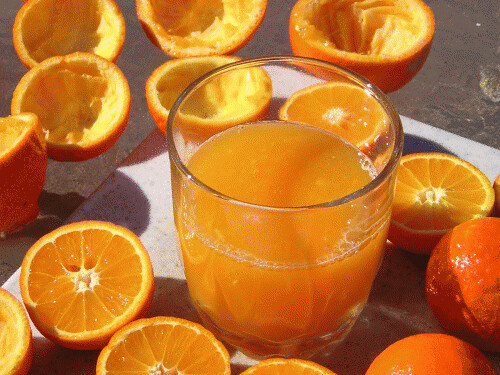The image features a smaller, round glass filled about two-thirds to three-quarters full with freshly squeezed orange juice, situated on a white-pinkish tabletop against a gray background. Surrounding the glass are various orange segments and remnants, meticulously arranged. Noticeably, six hollowed-out orange halves with their pulp entirely scooped out are spread around the upper portion of the scene, resembling empty orange rinds. In contrast, in front of the glass, there are seven or eight orange slices that have been halved but retain their juicy pulp. Additionally, in the lower right corner of the image, several whole, unpeeled oranges are conspicuously placed. The setting is bathed in direct sunlight, casting distinct shadows across the surface, suggesting a well-lit environment, potentially outdoors or near a large light source.